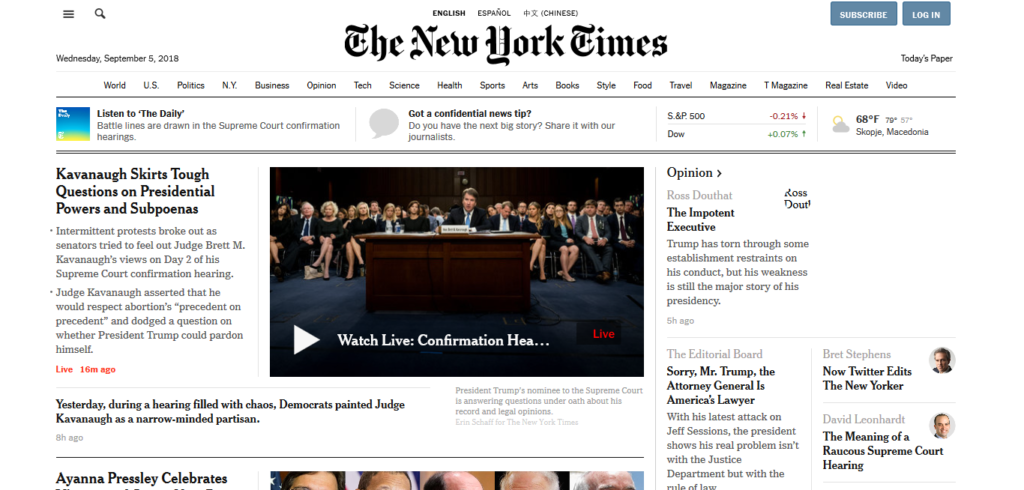The New York Times homepage as it appeared on Wednesday, September 5th, 2018, features a clean layout designed for easy navigation. At the very top, users can choose their language preference from options including English, Spanish, and Chinese. Next to this, on the left, the iconic triple-bar menu icon sits beside a search icon. To the right, prominent blue buttons invite visitors to 'Subscribe' or 'Log In.'

Below this header is the main navigation bar with the New York Times logo on the left and a 'Today's Paper' link on the right. The navigation menu allows readers to explore various news categories such as World, U.S., Politics, N.Y., Business, Opinion, Tech, Science, Health, Sports, Arts, Books, Style, Food, Travel, Magazine, T Magazine, Real Estate, and Video.

Beneath the navigation bar, a banner prompts readers to listen to 'The Daily.' Featured prominently is a headline about the Supreme Court confirmation hearings: "Battle lines are drawn in the Supreme Court confirmation hearings." Adjacent to this is a notice encouraging users to share confidential news tips or potential big stories with the journalists.

To the right of these notices, a stock ticker provides real-time financial updates, and next to it, a weather widget gives current conditions. The main content area features various articles from the day. A large video-linked story occupies the left side, inviting engagement through multimedia. To the right, an opinion piece by the editorial board stands out among several additional articles, predominantly focusing on political news.

The user interface balances informative content with interactive elements, maintaining a primarily black and white color scheme that emphasizes readability and a straightforward user experience.